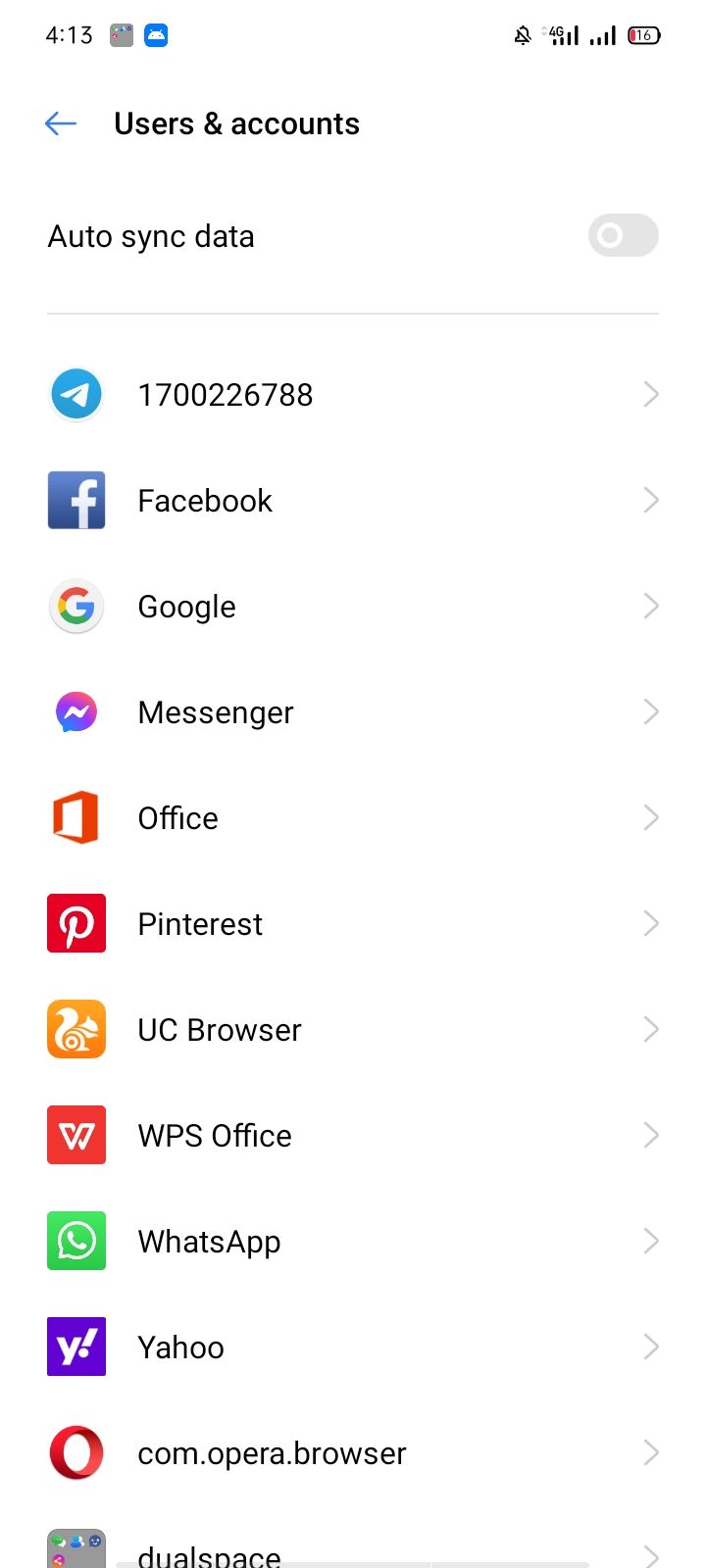The screenshot captures a "User and Accounts" settings screen on a cell phone. At the top, the title "User and Accounts" is displayed on the upper left-hand side, accompanied by a blue back arrow to its left. Directly underneath, the setting for "Auto-sync data" appears on the left side of the screen with a toggle switch on the right. The toggle is currently grayed out, indicating that it is in the "off" position. Following this setting, a thin gray separator line demarcates the section. Below the separator, a vertical list of accounts associated with the phone is presented. The list includes:

1. 1700226788
2. Facebook
3. Google
4. Messenger
5. Office
6. Pinterest
7. UC Browser
8. WPS Office
9. WhatsApp
10. Yahoo
11. com.opera.browser
12. Dual Space